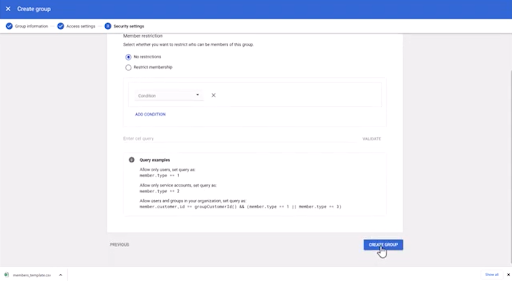This image is a blurry screenshot, making it challenging to discern specific details. It seems to depict a web interface for creating a group. At the top, there is a blue banner featuring an 'X' icon for closing the window and the text "Create Group." Below this banner, a white bar with three options is visible, each marked with a blue circle and a check mark, though the text details are unclear due to the blur.

The middle section of the image has a light reddish-gray background featuring a prominent white box. This box appears to contain questions, selectable toggle options, and a dropdown menu, all of which are indistinct because of the poor image quality. Further below, there is additional content that seems to provide some form of information, although it too is unreadable.

At the bottom of the image, two buttons are visible: an unselected one labeled "Previous" and a blue one labeled "Create Group," which is highlighted by a hovering pointer. Additionally, there is a status banner at the very bottom of the image, which seems to indicate a single page, but its precise contents are also obscured due to the blurriness.